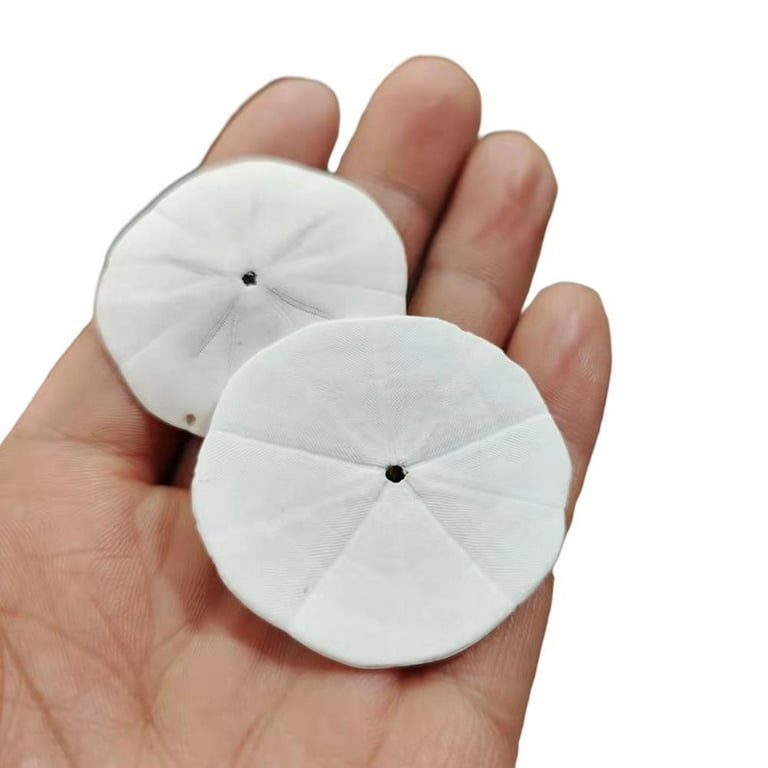This close-up image features a detailed view of a left hand set against a completely white background, holding two pristine white sand dollars. The hand, showcasing the four fingers and part of the palm, positions the sand dollars diagonally across the fingers, from the index to the pinky finger. The larger sand dollar sits atop the smaller one, each exhibiting intricate vein-like ribbing and complete, undamaged forms. The top sand dollar, which is slightly bigger, is oriented backside up with a central hole, while the smaller one beneath it is face up, revealing its artistic design. Both sand dollars are in excellent condition, with the bottom one also displaying a small hole near its edge, hinting at a place for a chain or string.